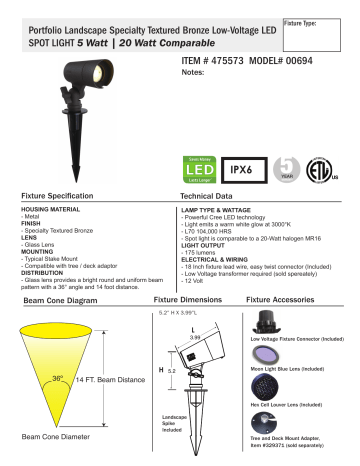**Detailed Caption:**

This image showcases a listing for the "Portfolio Landscape Specially Textured Bronze Low-Voltage LED Spotlight." The spotlight, which is black in color, is characterized by its 5-watt power usage, making it comparable to a 20-watt traditional spotlight. 

To the right of the spotlight image, the item number and model number are displayed, followed by a section for notes. Directly beneath this, a green box labeled "LED" indicates that this is an LED product, while a black-outlined box marked "IPX6" signifies its water resistance rating.

Additionally, there are two circles: one labeled "5-" with a partially obscured text and another stating "ETV." 

Below the spotlight image on the left side, detailed fixture specifications are provided. On the right side, technical details are listed, including lamp type, wattage, light output, and information regarding electrical and wiring requirements.

At the bottom of the image, there are three distinct boxes from left to right:

1. A "Beam Cone Diagram" box with a highlighted yellow diagram illustrating the light dispersion pattern.
2. A central box containing a detailed diagram of the spotlight itself, including dimensions.
3. A "Features" box on the right that lists the key attributes of the spotlight, although the text is too small to be legible.

This comprehensive layout provides a detailed overview of the product, specifications, and technical details, offering potential buyers thorough insight into the spotlight's features and capabilities.